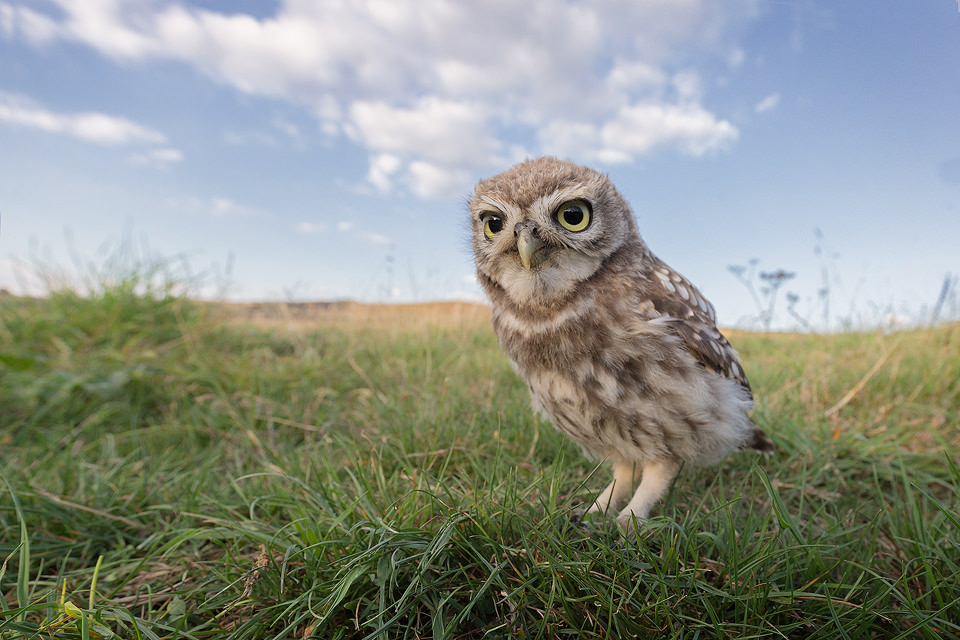The image is a color photograph in landscape orientation, capturing a young owlet standing in a grassy field. The scene depicts a clear blue sky with some light gray clouds occupying the top half of the frame, indicating a pleasant day. In contrast, the bottom half showcases a rich green grassy area interspersed with patches of brown, giving a natural, untended look to the open field setting.

Positioned slightly to the right of the center, the owlet is the focal point of the image. This baby owl features a speckled coat of brown and white feathers, with lighter shades around its eyes, neck, and stomach, and slightly darker wings. Its round, gold irises are accentuated by yellowish rings, giving it an expressive gaze. The owlet's thick legs are visible as it stands in a tuft of grass, facing slightly left and gazing somewhat upwards toward the viewer. The photograph embodies a style of representational realism, capturing the charming details of this young owl in its natural habitat.